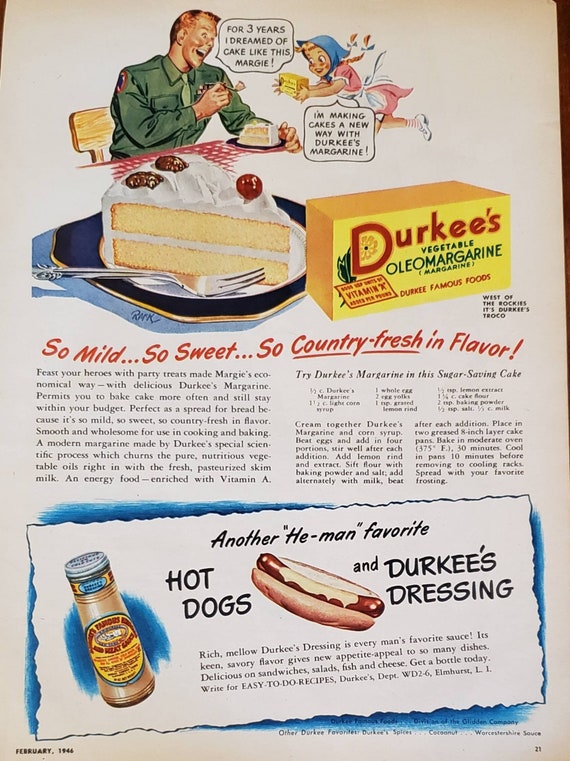This vintage magazine advertisement from February 1946 promotes Durkee's Vegetable Margarine, highlighting its versatility and flavor. At the top, a cartoonish image shows a man in military attire exclaiming, "For three years I dreamed of a cake like this, Margie." A joyful young girl, running towards him with a package of Durkee's Margarine, responds, "I'm making cakes a new way with Durkee's Margarine." Below this, the ad emphasizes the product’s qualities with the text, "So mild, so sweet, so country fresh in flavor," flowing gracefully in red. Accompanying the main text is a mouth-watering image of a slice of cake adorned with white frosting and fruit, presented on a black-trimmed square plate with a silver fork. The ad also features other food items, including a bottle of Durkee's dressing and a hot dog topped with this savory sauce, showcasing its appeal with the tagline, "Another He-Man favorite, hot dogs and Durkee's dressing." This rich, mellow dressing is touted as a man’s favorite, perfect for sandwiches, salads, fish, and cheese, promising to add keen, savory flavor to countless dishes. An appealing package of Durkee's Margarine is also prominently displayed, completing the nostalgic and appetizing scene.